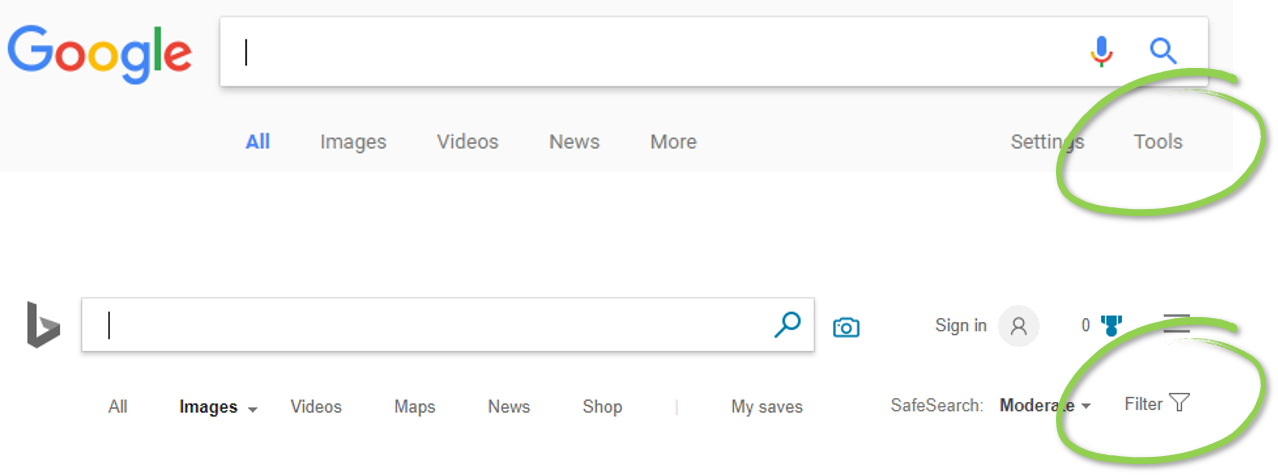The image depicts two distinct search bars set against a white background. The first search bar belongs to Google, identifiable by its colorful logo: the letter "G" in blue, followed by red, orange, blue, green, and the final "E" in red. This search bar features a text input box with a microphone icon and a magnifying glass symbol to its right. Below the search bar, there's a horizontal menu with the following options in blue and black text respectively: "All," "Images," "Videos," "News," and "More." On the right side of this menu are "Settings" and "Tools," with "Tools" highlighted using a green circle. 

The second search bar presents a different interface. It has an unfamiliar symbol to its left, resembling a folded-over triangle that points downward, then curls upward and slightly to the left. This search bar is shorter and includes a magnifying glass icon alongside a camera icon for visual searches. It also features options such as "Sign In" and a user figure icon, followed by additional elements on the right. Underneath, the navigation options mirrored below the search bar include: "All," "Images" (bolded), "Videos," "Maps," "News," "Shop," "My Saves," "Safe Search," and "Moderate." Here, the "Filter" option is circled with a green marker.

In summary, the image showcases two different search bar designs, one from Google and another with a different, unfamiliar symbol, both detailed with various navigation and tool options highlighted and circled in green.